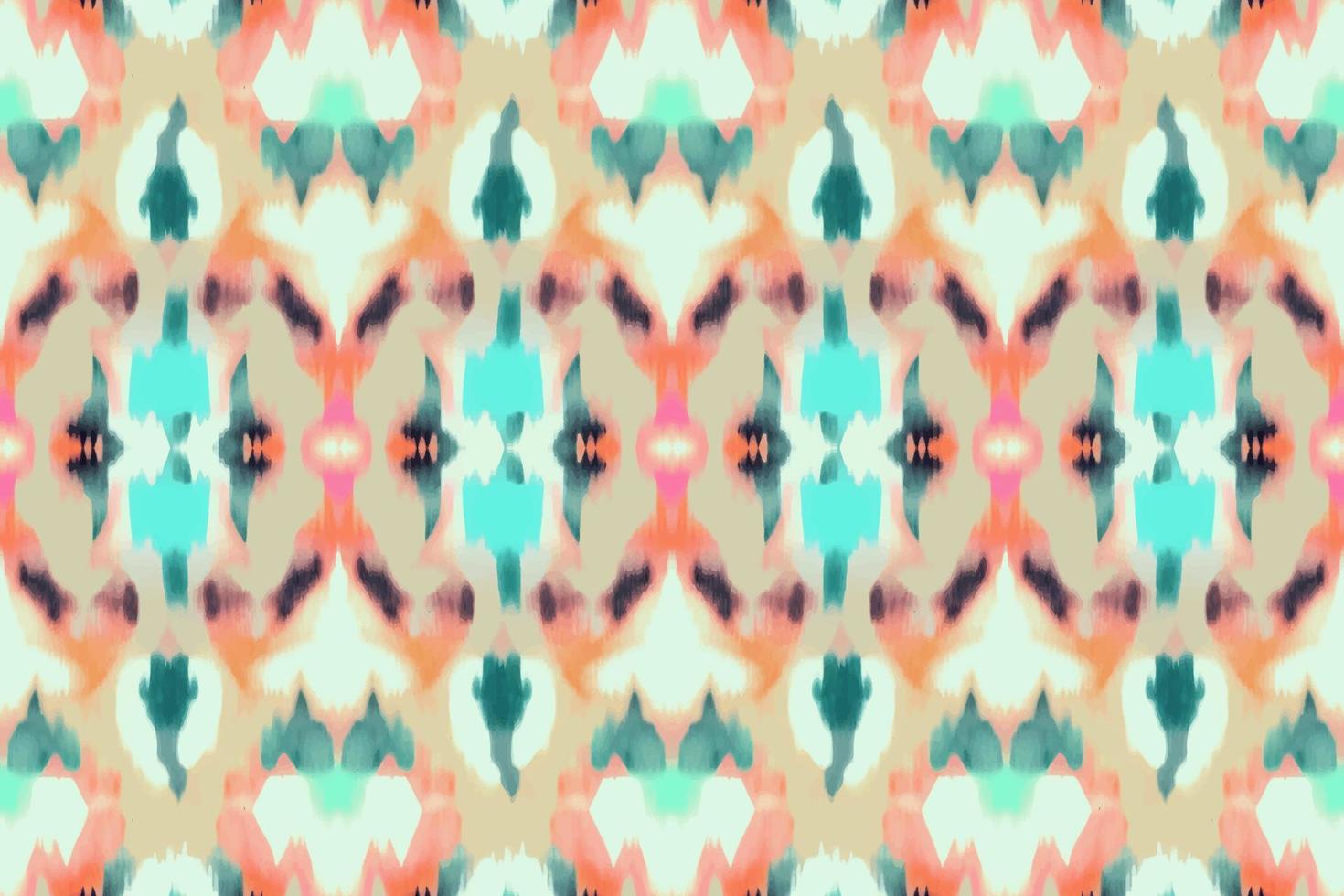The image is an abstract painting featuring a blurry, yet consistent repeating pattern, reminiscent of a psychological Rorschach test. The painting is horizontal with a cream-colored background and various intricate shapes and colors. The dominant colors include orange, green, teal blue, pink, beige, and white, with dark purples appearing prominently in the middle section from left to right.

At the top, there is a row of shapes resembling demonic cow heads with horns, characterized by white and dark eye areas, orange floppy ears, and pink tubular connections. This top pattern creates a visually complex design. Beneath this, the next row features an orange flame-like shape with white centers, green circles near the base, and two dark green blobs resembling bird tails, extending horizontally. This row contains five of these flame-like patterns.

Further down, a row of white circles with tall green shapes in their centers spans across the image, followed by a row of alien-like heads with ram's horns and large black eyes, depicted five times across. The next row includes four blue rounded rectangles with black bird-like shapes on both sides.

Within the middle section, patterns that resemble birds flying from a top-down perspective become prominent, giving a sense of motion. There are also heart-like shapes and figures that appear like ducks standing on their back feet, reaching towards the sky, seen towards the top left and repeating across and upside down at the bottom.

This brilliantly colorful and intricate pattern repeats throughout the painting, creating a mesmerizing kaleidoscope effect that draws the viewer into its abstract and almost otherworldly design.